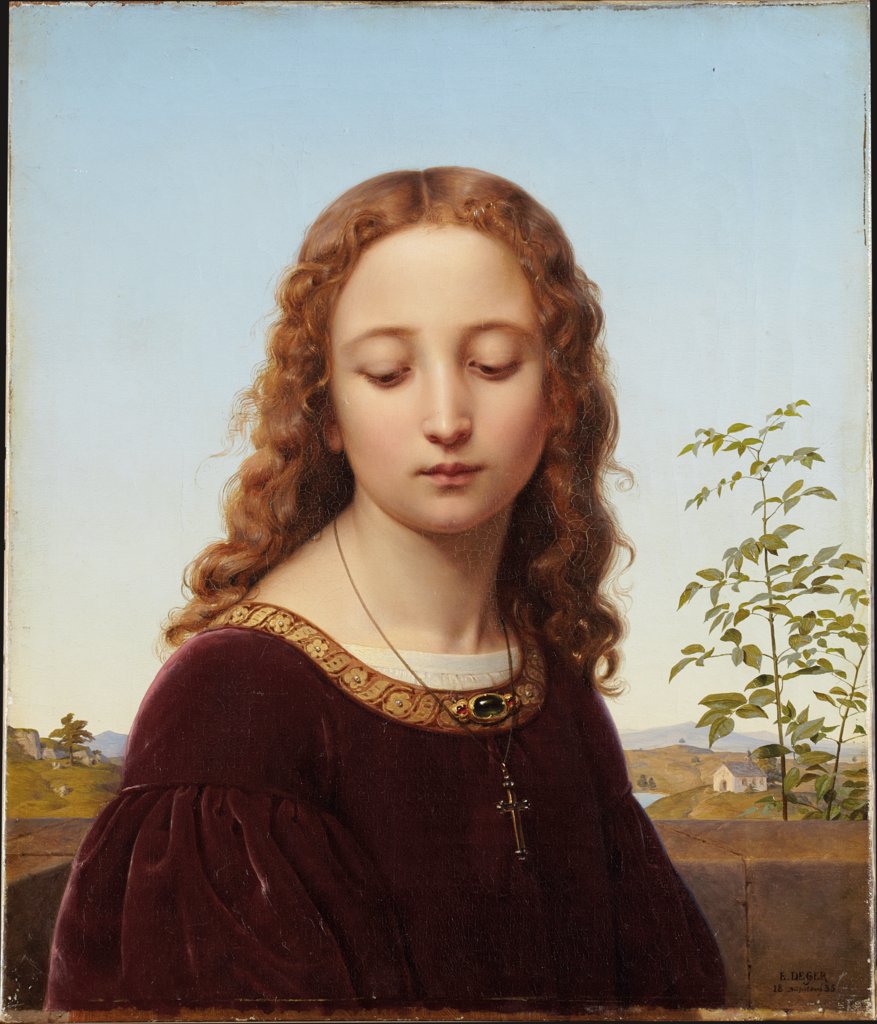This image depicts an oil painting in the style of the Renaissance, featuring a fair-skinned woman with long, curly, light brown to reddish hair that cascades over her shoulders, parted in the middle. She is dressed in a velvety red gown adorned with gold trim, with her head tilted downwards, eyes looking toward the right, and a closed mouth, giving her a somber, downcast expression. The woman wears a prominent necklace with a cross pendant hanging over her chest. The backdrop presents a serene blue sky, which fades to a whitish hue at the center, complemented by brown hills and distant mountains on the left. On the right side, branches with leaves add detail, and behind them stands a white house with a gray roof. Additionally, there is a hint of a water body visible near the building, enhancing the landscape's serene ambiance.